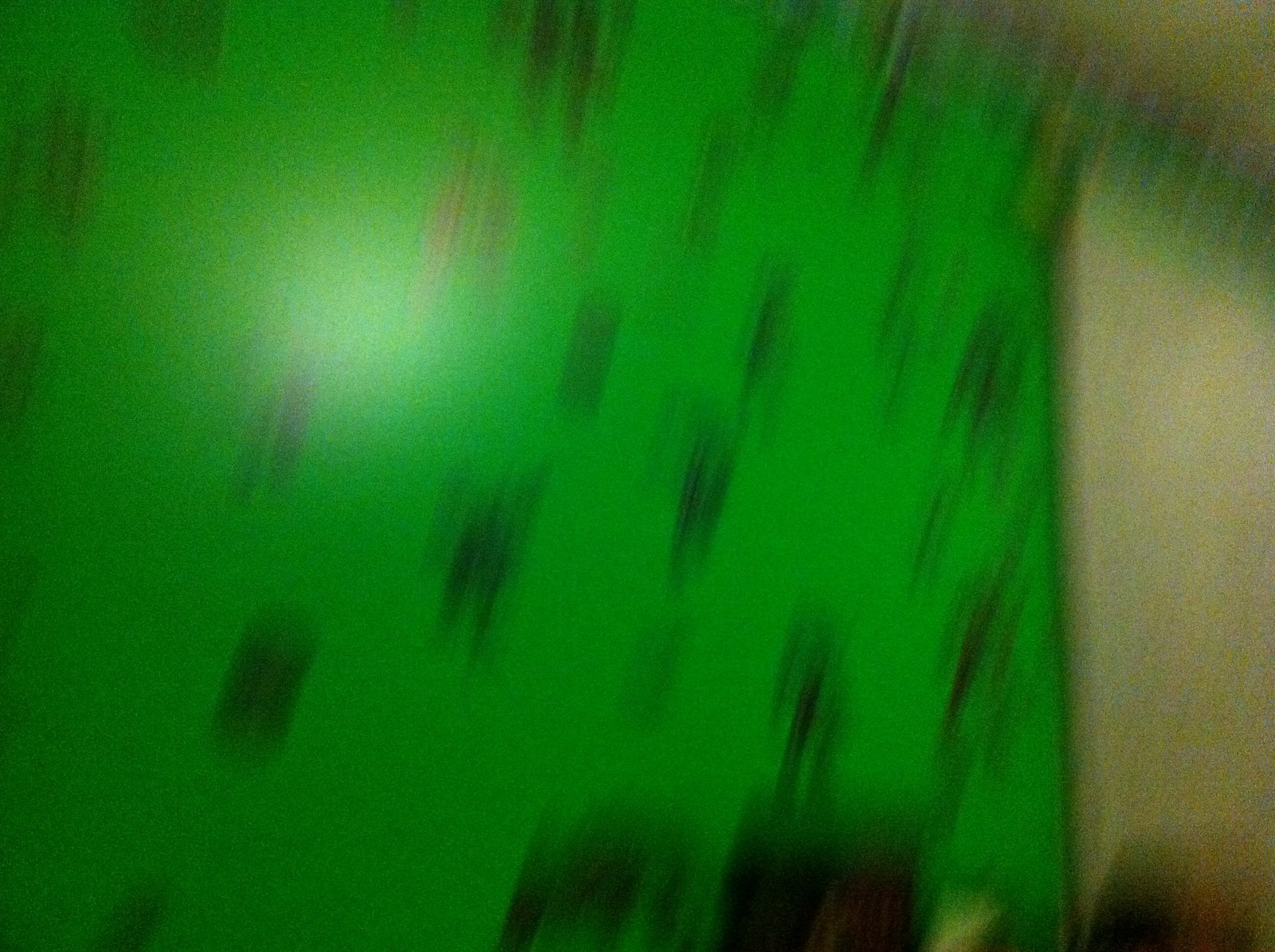A heavily distorted and blurry photograph showcases a wall divided into two distinct sections. The left side features a lime green backdrop with ambiguous black graphics that resemble the silhouettes of soldiers or figures, though the blurriness makes them indiscernible. The right side of the image presents a tan wall, separated from the lime green section by a horizontal border comprised of shades of yellow, green, and black. The lower part of the photograph is obscured by an array of color distortions in black, yellow, and faint hints of red. Overall, the image is characterized by its grainy quality and significant white distortion that obscures finer details.